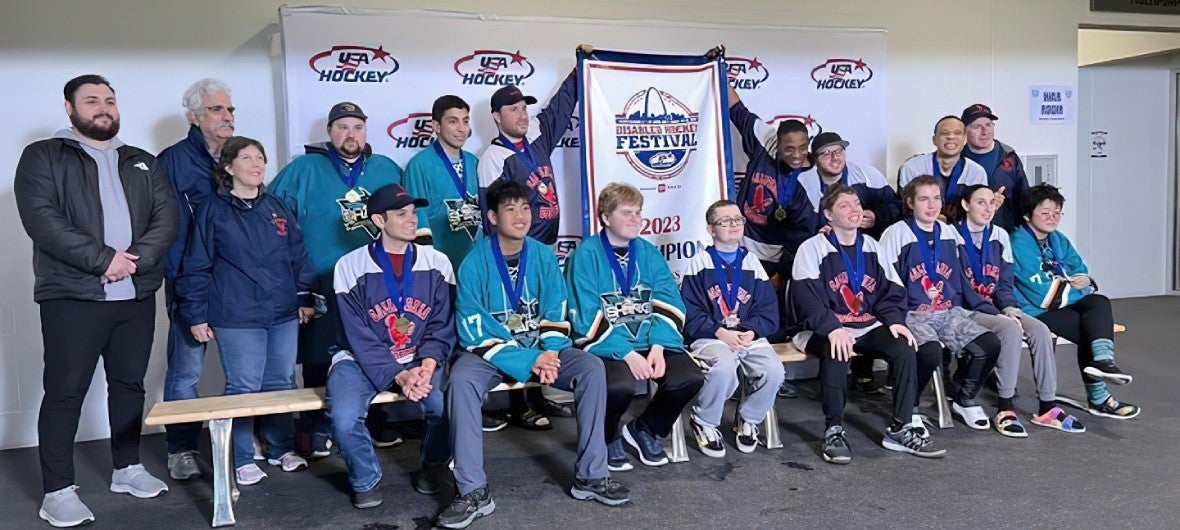This detailed photograph captures a jubilant moment at the Disabled Hockey Festival in 2023, featuring the winning championship team seated on a bench. Prominently displayed in the foreground are eight young athletes, ranging in apparent age from 15 to 17, each proudly wearing a medal around their neck. The team is a mix of mostly young men and a few women, with varying, sometimes visible disabilities, all exuding happiness and pride. Some athletes are clad in teal blue jerseys with black and white stripes, while others don navy blue jerseys. A large banner held aloft behind them announces "Disabled Hockey Festival 2023 Champions," with a larger "USA Hockey" banner in white with blue print and a red star partially visible in the background. Standing behind the team, a group of smiling adults, possibly parents and coaches, contributes to the celebratory atmosphere in this indoor setting against a white wall.